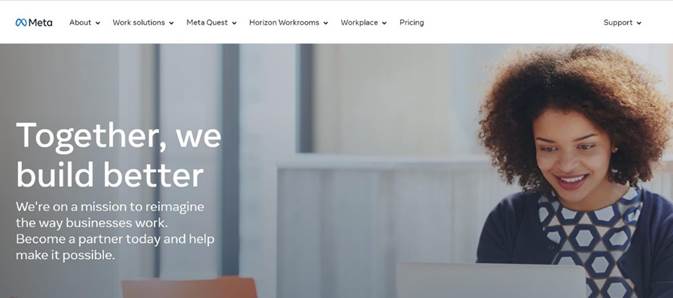The image features a primarily blue background and at the top of the image, there is a white box adorned with a small blue insignia resembling butterfly wings next to the word "Meta." Below this, there are several navigational elements including buttons with arrows labeled "Work Solutions," "Meta Quest," "Horizon Workrooms," "Workplace," "Pricing," and "Support."

In the center-left of the image, there is a prominent piece of brown paper that contains a motivational message: "Together we build better. We're on a mission to reimagine the way businesses work. Become a partner today and help make it possible."

To the right of this text, the image shows a young lady with curly hair wearing a blue jacket over a blue and white top. She is seated at a white computer, appearing focused and engaged. The entire scene is set against a blue wall and door, creating a cohesive and professional atmosphere.